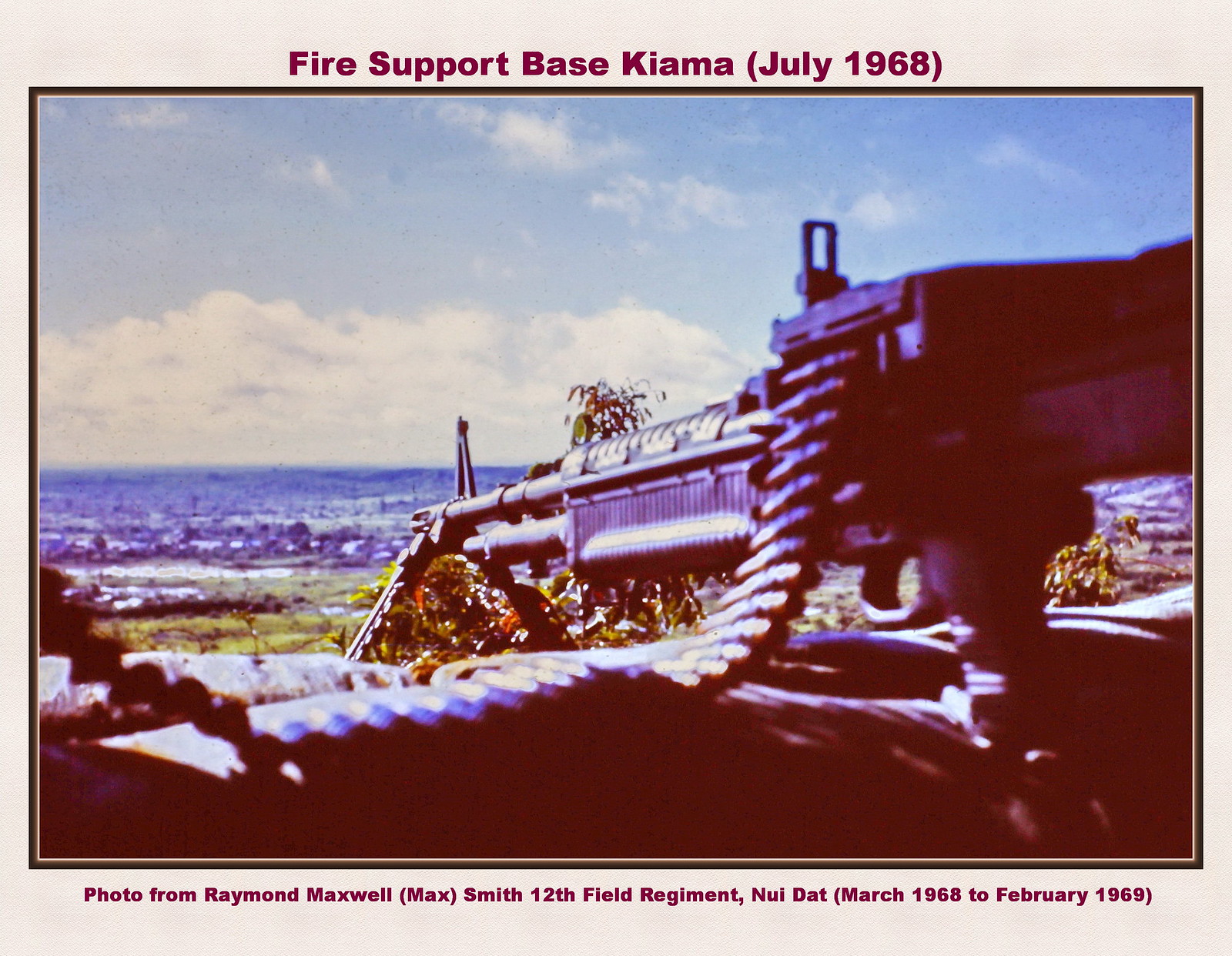The image depicts a scene from the Vietnam War in 1968, labeled at the top with "Fire Support Base Kiyama, July 1968" in maroon font. A mounted machine gun dominates the foreground, its long artillery belt hanging to the side with approximately 50 large bullets visible. The gun is directed towards a distant field, further characterized by a waterfront area with palm trees, blue skies, fluffy white clouds, and a small mountain range on the horizon. Below this scenic backdrop, piping structures and possible barracks are faintly discernible. The photo features a dark border, and the bottom credits read: "Photo from Raymond Maxwell, Max Smith, 12th Field Regiment, Nui Dot, March 1968 to February 1969."